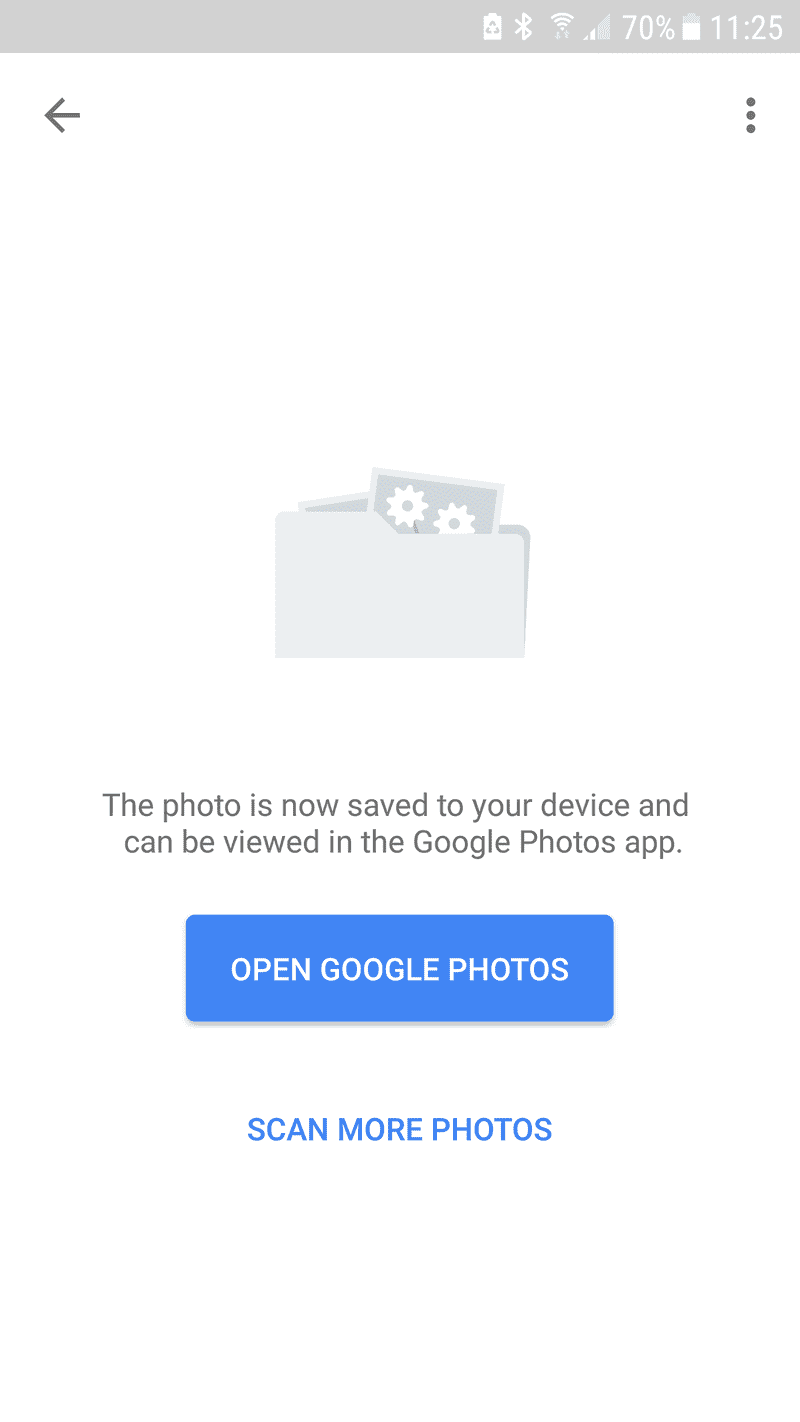This image is a mobile screenshot with a vertically oriented, minimalist design. At the very top, there is a light gray status bar containing several white icons aligned from left to right. The first icon resembles a battery with a small triangle inside, indicating a 70% charge. This is followed by the Bluetooth symbol, the Wi-Fi symbol, and signal bars with two out of three bars filled. To the far right, the time is displayed as 11:25.

Beneath the status bar, the background is completely white. On the left-hand side, there is a black back arrow, while on the right-hand side, there are three vertical dots indicating a menu option. In the center of the screen, a gray icon is prominently displayed, featuring a cartoony design of a slightly open gray folder containing two photographs. The photographs are dark gray with light gray borders; one of them, more visible than the other, displays two white gear symbols.

Underneath this icon, black text reads, "The photo is now saved to your device and can be viewed in the Google Photos app." Below the text, a blue button labeled "Open Google Photos" is present, followed by another option labeled "Scan More Photos."